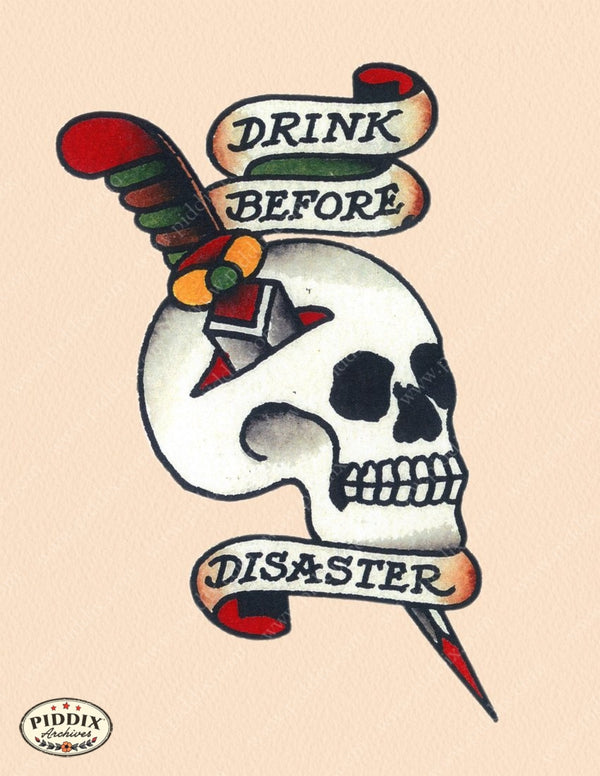The illustration features a detailed, playful skull facing right, set against a peach background. A colorful knife with a red tip pierces through the skull, whose closed teeth and blacked-out eye and nose sockets add to its stylized charm. The knife handle is elaborately designed with alternating red and green colors, a golden medallion, and an emerald green stone at its center. A bold ribbon-like banner winds around the skull, inscribed with the phrase "Drink Before Disaster." The ribbon is cream-colored with shaded edges, and its underside is red. In the lower left-hand corner, an oval with three stars and a small flower logo bears the text "Piddocks Archives," indicating the creator of this vibrant, tattoo-style artwork.